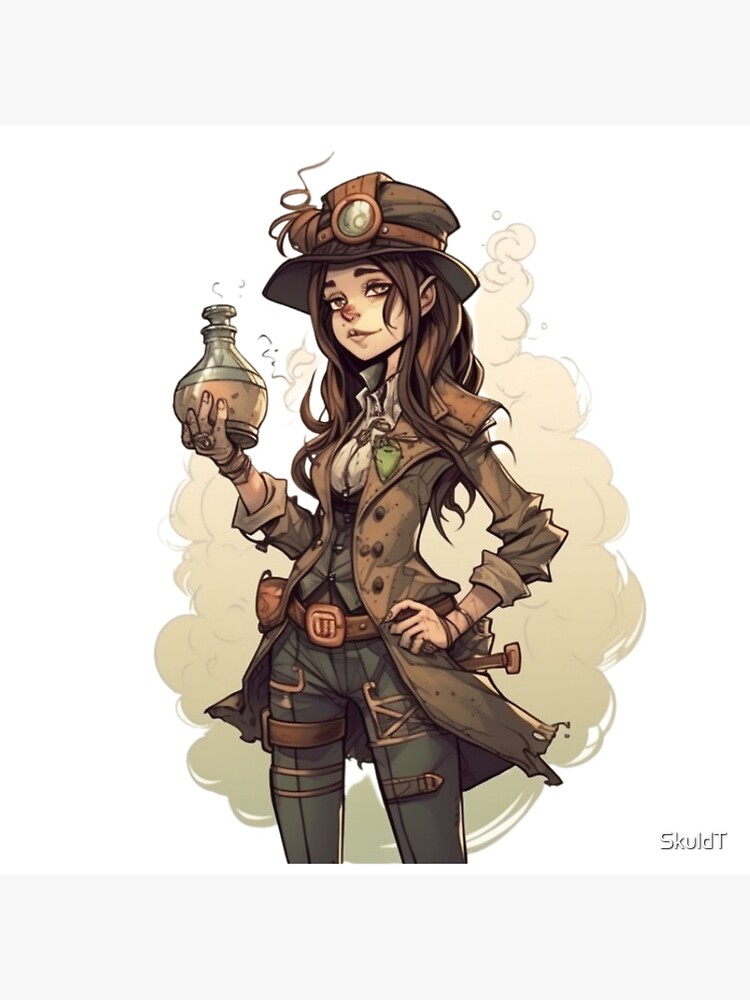This detailed painting depicts a young woman of European descent dressed in steampunk fashion. The background is white, highlighting the intricate details of her attire and character. The artist, whose name "Skuldt" is inscribed in the bottom right corner, has masterfully captured a rugged yet elegant essence.

The woman has long brown hair that cascades down to her torso and pointed ears that give her a slightly otherworldly appearance. She wears a brown three-quarter length overcoat with three visible buttons on the side, under which she sports a vest and an off-white shirt. A brown belt with three lines on the buckle cinches her waist, complemented by a corset that adds structure to her ensemble.

Her outfit features numerous steampunk embellishments, including harnesses and straps around her pant legs—three on the right leg and two on the left. The pants themselves are dark green, harmonizing with the overall earthy tones of her attire. On her head, she wears a brown top hat adorned with a wooden band and a light-colored medallion in the center.

The woman’s right hand holds a goblet-style bottle with a stopper, containing a yellowish liquid, while her left hand rests confidently on her hip. A puff of smoke rises behind her, suggesting the magical, genie-like qualities of the bottle. Adding a final touch of detail, she wears a ring on her finger, accentuating her steampunk aesthetic.

The image is styled with a blend of magazine and anime colorings, contributing to the vibrant, animated feel of the artwork.